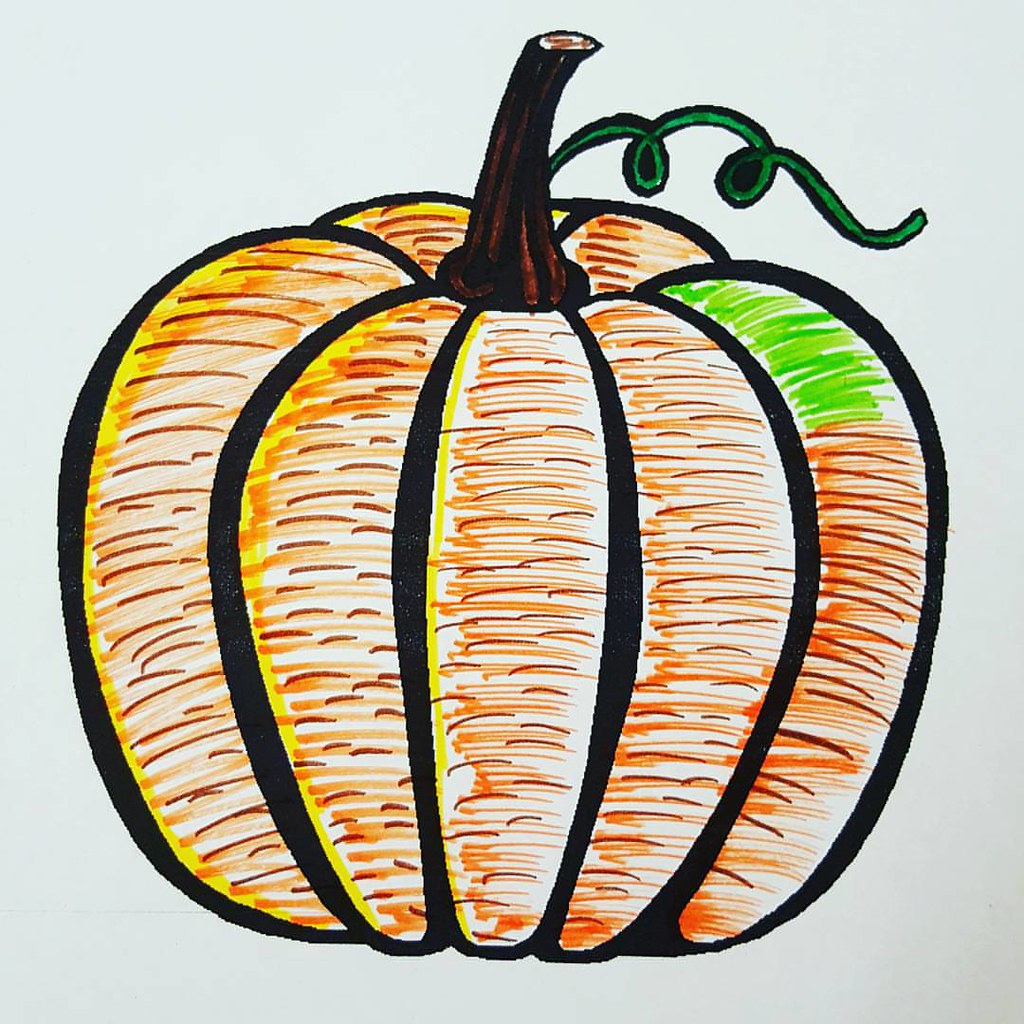This image showcases a highly detailed and vibrant artwork of a pumpkin, occupying the majority of a square canvas. The pumpkin is meticulously outlined in a thick black marker, clearly defining its round shape and segmented flesh with vertical lines. The pumpkin is predominantly colored using densely drawn horizontal lines in varying shades of orange, yellow, and deep red, with a hint of brownish markings and a small green section adding depth and texture. At the top, a dark brown and black stem extends outward, accompanied by a green, curly vine. The background offers a muted contrast, featuring predominantly medium to dark gray tones, creating a subdued, almost monochromatic backdrop that highlights the vivid colors of the pumpkin.